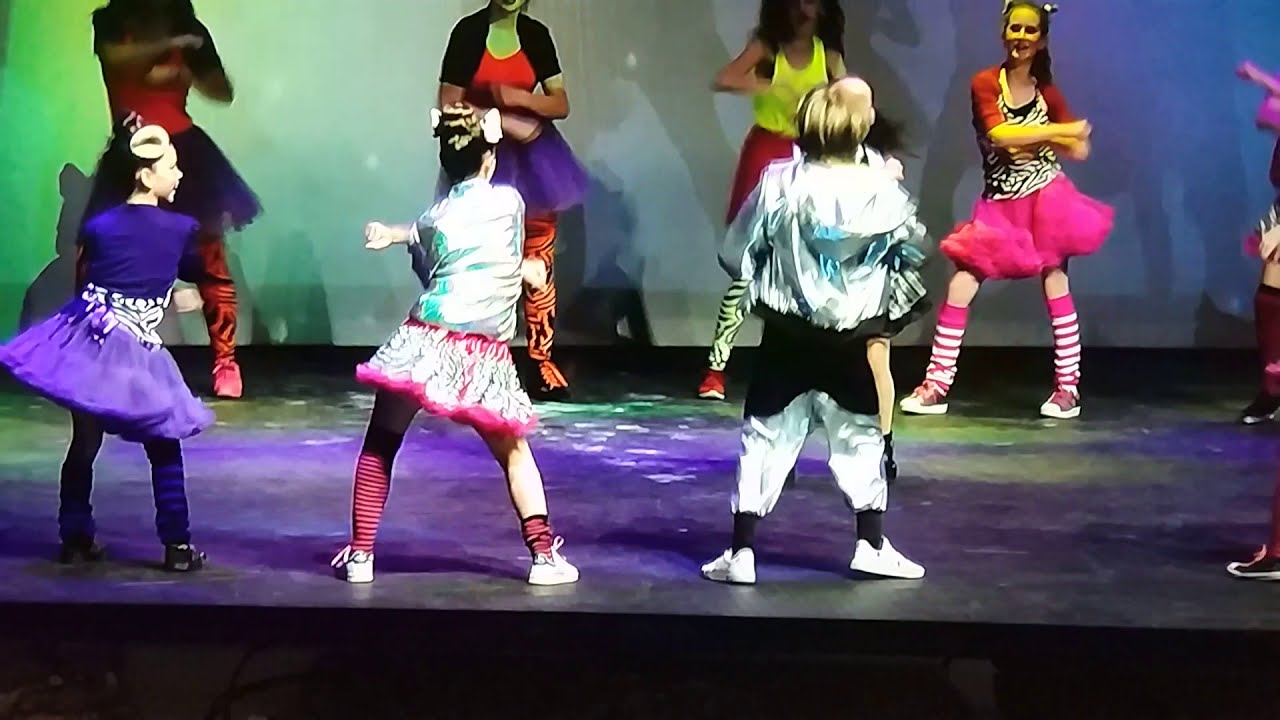The photograph captures a vibrant dance performance on an elevated, colorfully lit stage with green and purple lights that create a lively atmosphere. In the foreground, three children strike dynamic poses. The left child wears a blue top, a purple dress, and blue leggings. The center child dons a striking silver top paired with a silver and pink dress and red and white leggings. On the right, a child, possibly a boy, stands out in a complete silver ensemble with baggy pants, a shiny jacket, and black socks, showcasing blonde hair. 

In the background, a row of larger children, possibly adults, are fully engaged in synchronized dance moves, rotating their forearms around each other, their arms elegantly positioned in front. Their eclectic costumes feature tutus of varied colors—purple and pink skirts stand out—combined with blouses in shades of yellow, red, lime, black, and white. They sport multicolored leggings, adding a playful touch to the scene. The cohesive yet diverse costumes contribute to the overall festive and dynamic energy of the performance.